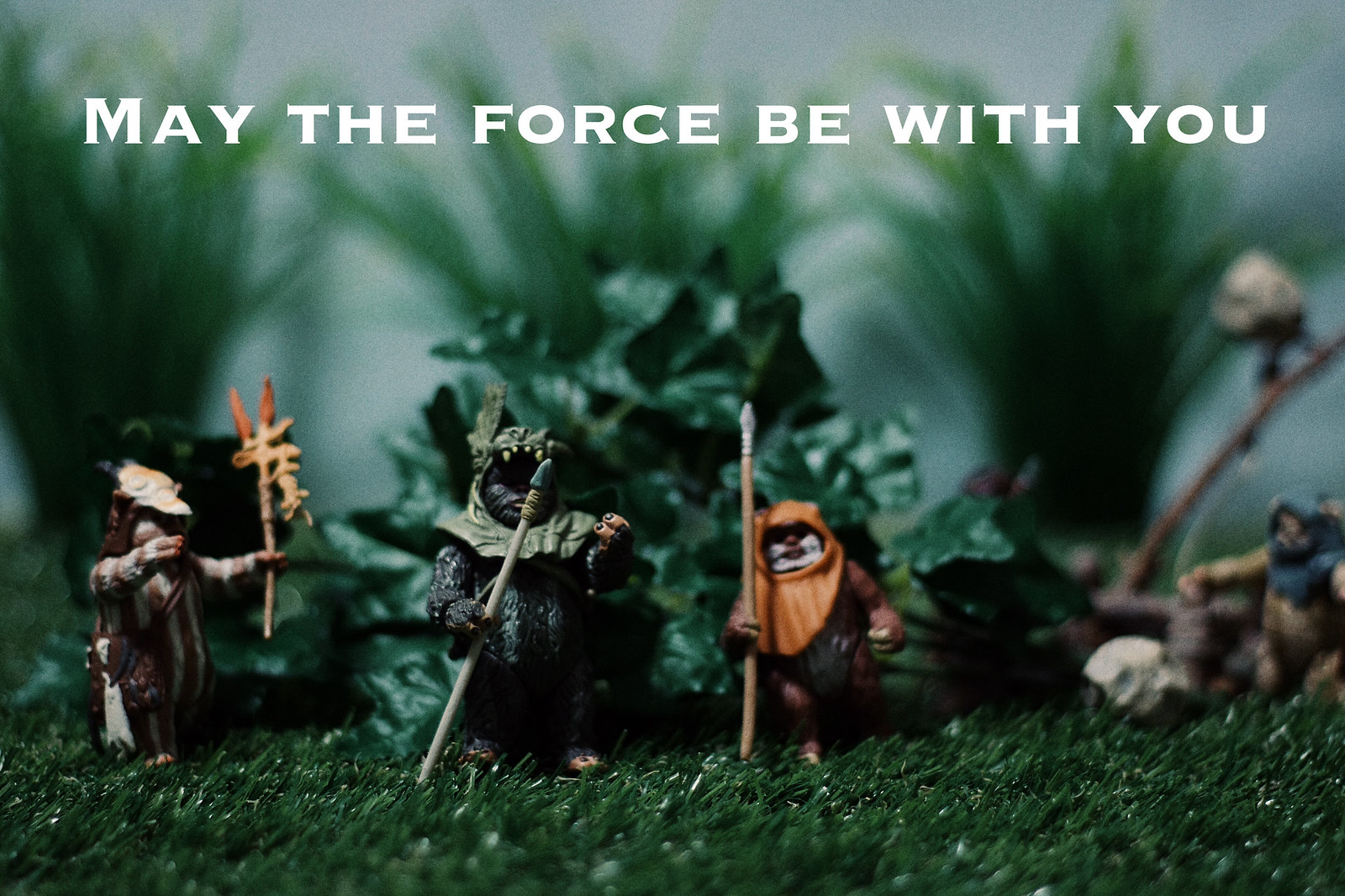This horizontally aligned rectangular image predominantly features shades of green and black, with bold, all-caps white text across the top that reads, "May the Force Be With You." The upper background showcases a blurred array of elongated plant leaves against a grayish haze. In the foreground, dark green, possibly artificial grass or astroturf serves as the base for a miniature diorama set. The scene includes four small figures resembling Ewoks, each adorned in their traditional attire. Centered is an Ewok equipped with a wood pole spear, brown with light brown accents. To its left is another Ewok-like figure, darker brown with a green hood. On the far left, a creature holds a weapon, while on the far right, a similarly brown creature with a blue hood is partially obscured by blur. The diorama meticulously recreates a scene reminiscent of the Star Wars universe, with the Ewoks standing out amid detailed foliage and atmospheric elements.